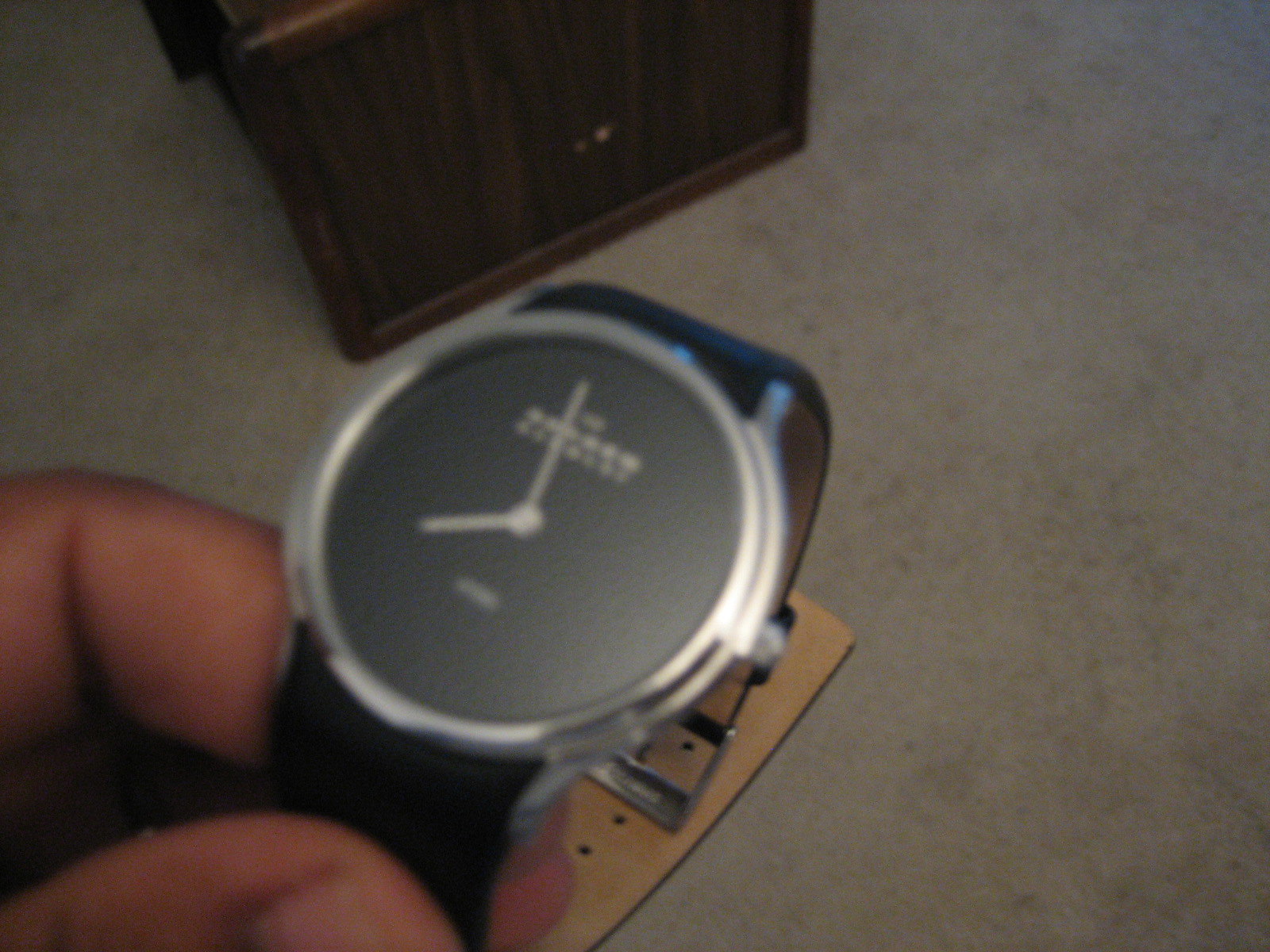The image depicts a close-up view of a hand holding a wristwatch. Only the thumb and index finger of the hand are visible, emerging from the bottom left corner of the frame, grasping the watch. The background shows a brown floor with variances in shade, some light and dark spots, and a piece of furniture partially visible. The watch occupies about a third of the image, extending from the left edge toward the center.

The wristwatch itself features a sleek black face devoid of numbers, giving it a minimalist appearance. The hour and minute hands are slender and white, while a small amount of writing is present at both the top and bottom of the watch face. Surrounding the face is a bright silver bezel. The band of the watch is black leather on the outer side, whereas the inner side is a light brownish color. Additionally, a metal buckle is attached at the end of the band.